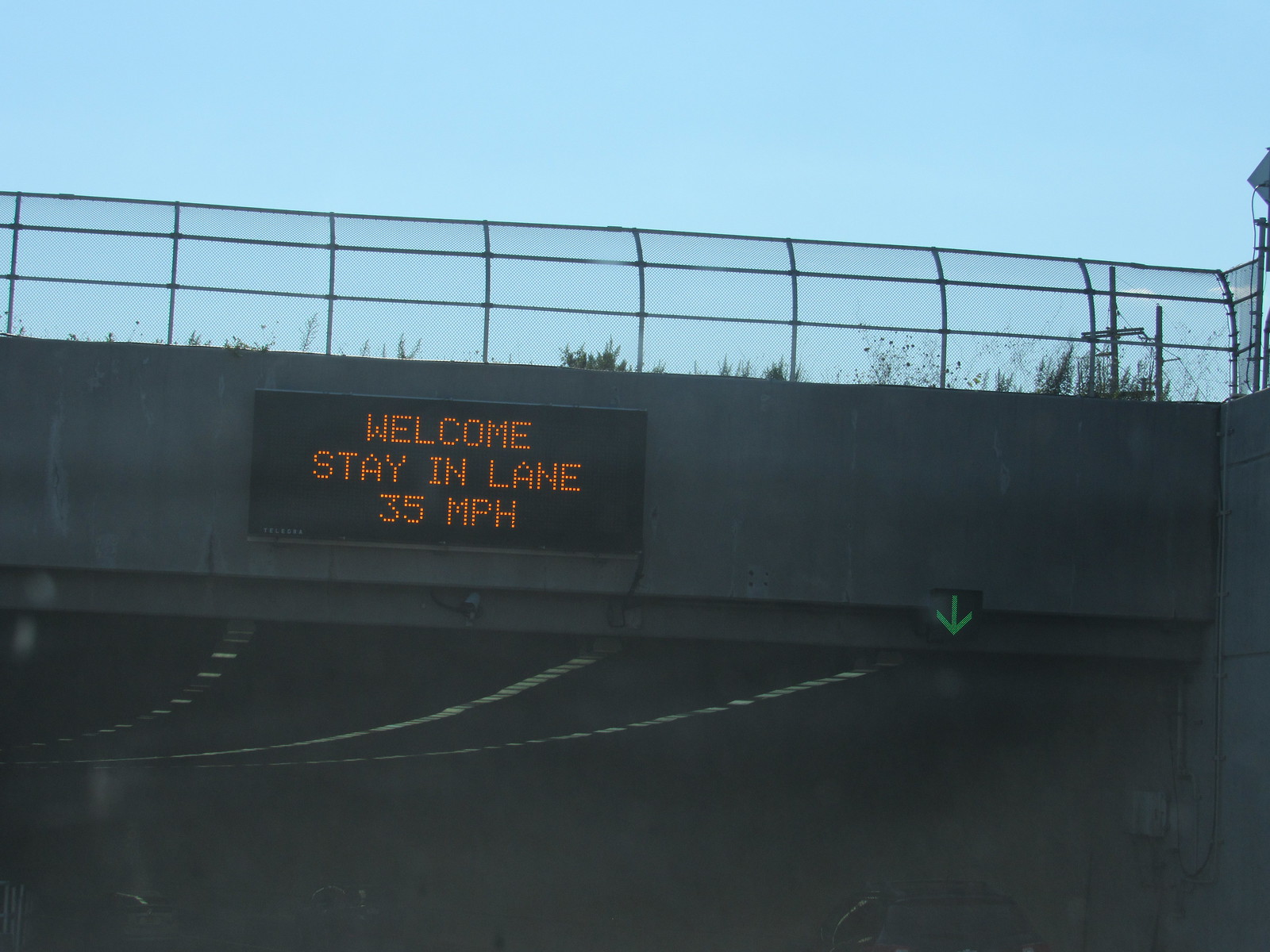The image showcases a modern overpass or tunnel set in an outdoor environment. Prominently displayed on the overpass is a black electronic sign, which is illuminated with amber-colored lights displaying a three-line message: "Welcome" on the top line, "Stay in Lane" in the middle, and "35 Miles Per Hour" at the bottom. Towards the bottom right of the sign, a green downward-pointing arrow is visible.

The tunnel beneath the overpass is lit by three rows of lights that extend inward, creating a sense of depth. Above the tunnel, there is a metal fence that stretches across the top, beyond which some small plants are visible. In the background, the clear blue sky provides a contrasting backdrop to the structure.